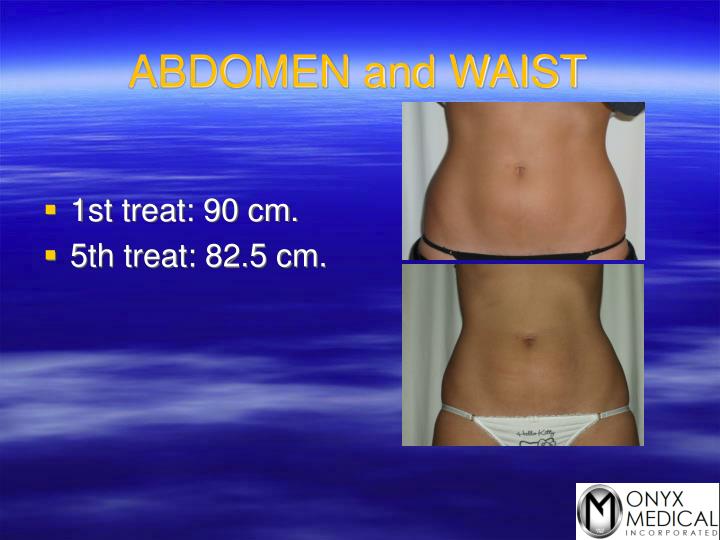The image depicts a PowerPoint slide with a blue and white textured background, resembling waves. At the top of the slide, there is a bold, yellow heading that reads "ABDOMEN AND WAIST." On the left side of the slide, there are two yellow bullet points with white text that state: "First Treat: 90cm" and "Fifth Treat: 82.5cm." To the right, there are two images stacked vertically, showing the waist of a woman before and after treatment. The top image displays a wider waist, while the bottom image shows a slimmer, more toned waist. At the bottom right corner of the slide, there is a logo for Monix Medical Incorporated, featuring a silver circle with a black "M" inside, and the company name written in black text against a white background, with "Incorporated" in a smaller font size.